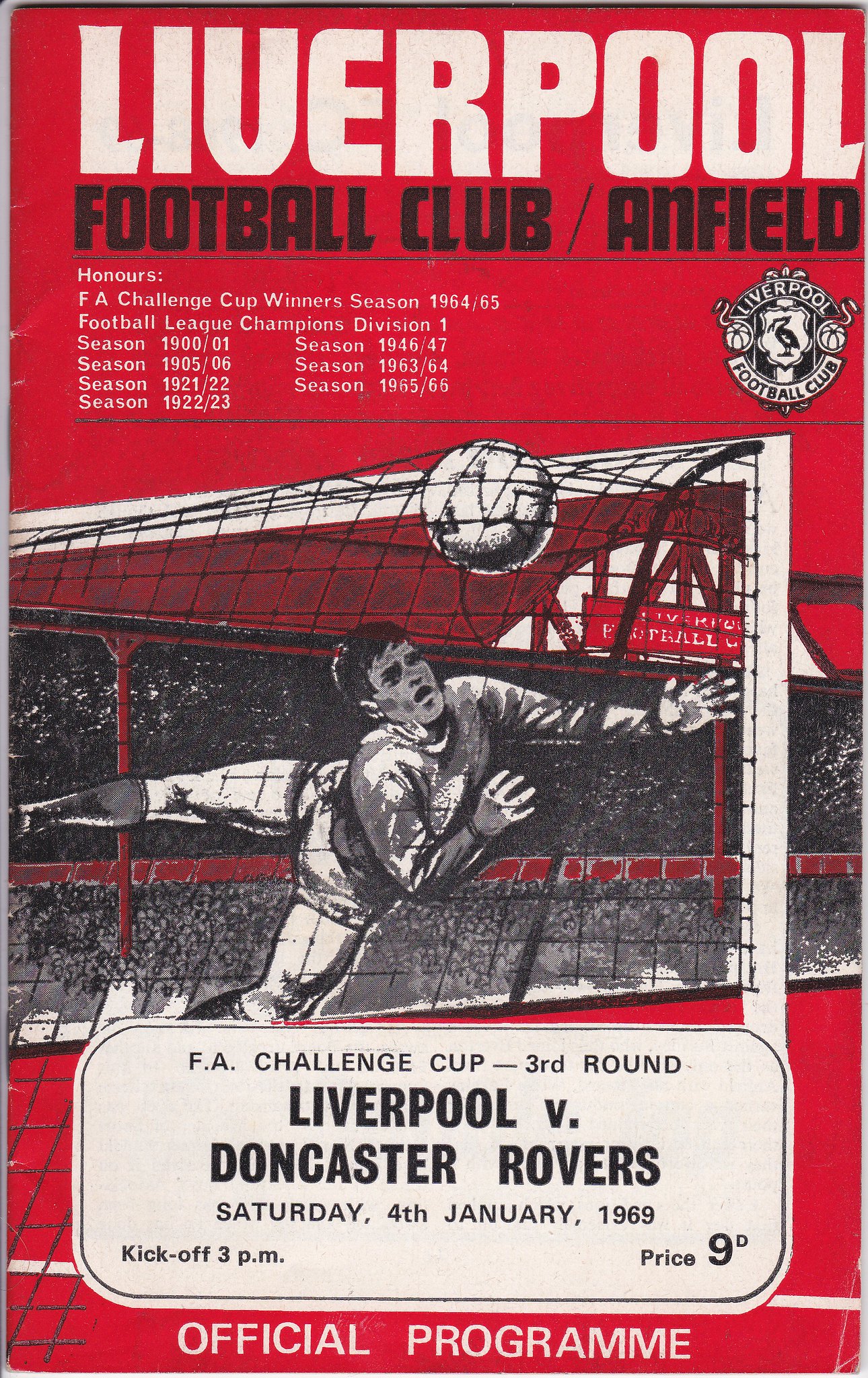This is an image of the official program cover handed out during the F.A. Challenge Cup Third Round match between Liverpool Football Club and Doncaster Rovers, held at Anfield on Saturday, January 4, 1969, with a kickoff at 3 p.m. Dominated by a striking red background, the program features large white fonts at the top reading "Liverpool Football Club Anfield," with a subheading listing various honors in smaller white text that includes their F.A. Challenge Cup win in the 1964/65 season and multiple Football League Championships. The upper right corner displays the Liverpool F.C. crest, depicting a crane within a shield-like design. Towards the center, a detailed pencil drawing captures a dramatic moment of a goalkeeper diving to save a ball that has just hit the net, set against a backdrop that includes a glimpse of a crowded stadium with audience stands and signboards. The bottom section of the program contains a white box with black text providing match details: "F.A. Challenge Cup Third Round, Liverpool vs. Doncaster Rovers, Saturday, 4th January 1969, kickoff 3 p.m.," followed by the price, $9.00. At the very bottom, a footnote in white text states "Official Program."